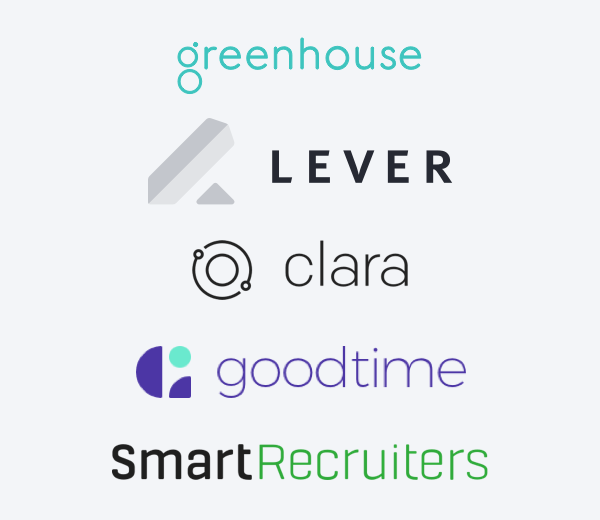The image features a large shaded gray square centered against a white backdrop, with white space extending uniformly on all sides. At the top center of the image, the word "greenhouse" appears in green, all in lowercase letters. Notably, the "G" is stylized using two circles, reminiscent of a binocular design, with a small dot above the top circle. Directly beneath it, the text "LEVER" is displayed in capital letters in black. 

To the left of the text, there is a 3-dimensional representation of a rectangle or box, rendered in shades of gray, with a subtle gray triangle beneath it, suggesting depth. Adjacent to this, the name "Clara" is written in small black letters. Accompanying this name is an illustrative black circle containing a smaller gray circle at its center, matching the gray background but distinctly outlined.

Further along, in small purple letters, the phrase "good time" is inscribed. Alongside this text is an emblem featuring a vertically aligned half-circle in purple, paired with a turquoise circle and complemented by an additional small quarter-circle in purple.

At the bottom portion of the image, the phrase "smart recruiters" is presented, with "smart" in black and "recruiters" in green, marking the conclusion of the textual elements.